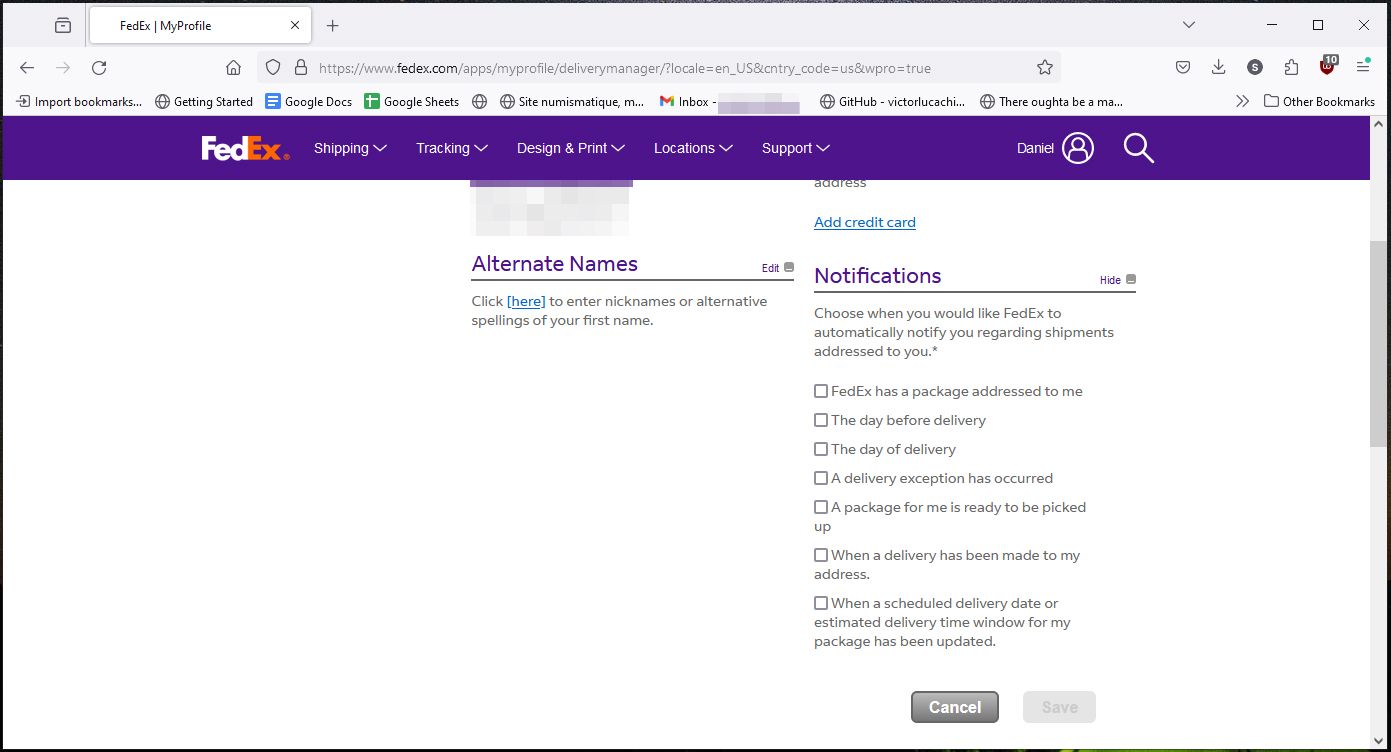This image displays a page from the FedEx website, specifically focusing on user account settings and notifications. The webpage features various tabs such as "Shipping," "Tracking," "Design & Print," "Locations," and "Support." An important detail includes the user's name, "Daniel," which is visible on the side, along with an option to enter a nickname or alternate spelling of the first name.

The notification settings section allows users to customize how they receive updates related to their packages. Users can opt to be notified for events such as:

- A day before delivery
- On the day of delivery
- If a delivery exception occurs
- When a package is ready for pickup
- When delivery is made to their address
- When the scheduled delivery date or estimated delivery time window is updated

The page concludes with two actionable buttons labeled "Cancel" and "Save," giving users the option to either discard or confirm their notification preferences.